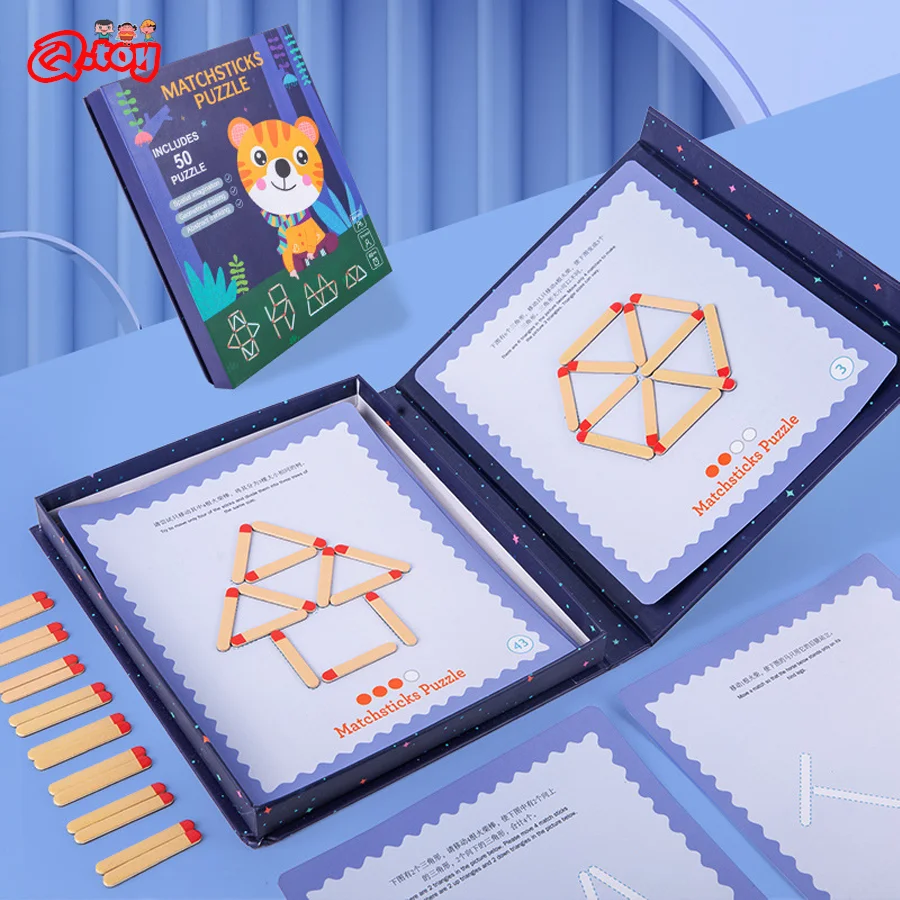This image is a promotional product photo for a children's matchstick puzzle book from Qtoy, displayed on a blue desk in a blue room with a blue curtain partly visible in the top left corner. The book's cover is a vibrant blue and green and features an orange cartoon tiger with reddish-orange stripes wearing an orange shirt. Notably, the top left corner of the cover shows the Qtoy logo in red text with three small character symbols above it. The book title, "Matchstick Puzzles," prominently states that it includes 50 puzzles.

In the foreground, the book is opened to display its puzzles. One page showcases a level 3 difficulty puzzle completed in the shape of a house, labeled on grayish-blue paper with a dark blue border, and a level 2 puzzle resembling the EXO K-pop band's hexagonal logo. Both pages contain captions in Korean (Hangul) with English subtitles below. Additional matchsticks, totaling eight pairs, are visible scattered around the scene, reinforcing the book's interactive element. The detailed matchstick arrangements provide patterns that can create various shapes, such as a wheel and a pizza, displayed across different levels of complexity. The comprehensive bilingual presentation enhances its appeal, ensuring engaging entertainment for children.